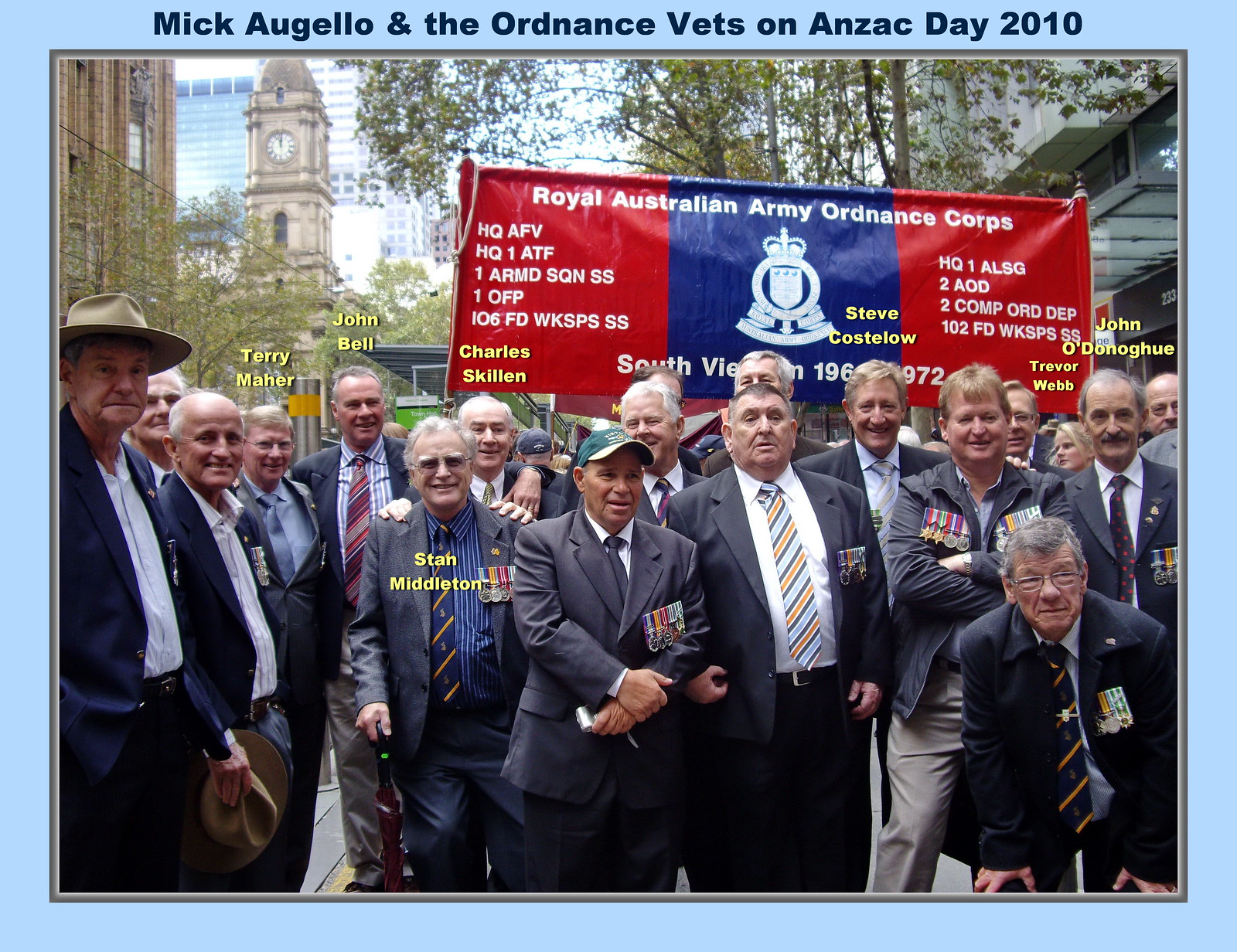This detailed photograph captures a group of elderly Caucasian men, all wearing suits adorned with war medals, commemorating Anzac Day in 2010. The men, including individuals named Terry Mayher, John Bell, Stan Middleton, Steve Costello, John O’Donohue, Trevor Webb, and Charles Skillen, stand in front of a red, white, and blue banner with the inscription, “Royal Australian Army Ordnance Corps.” The banner, featuring an Australian seal in the center, is positioned slightly behind the men. In the background, a skyline of buildings, including a clock tower and skyscrapers, as well as some trees, can be discerned. The scene is framed by a light blue border with the additional text at the top reading, “Mick Ogillow and the Ordnance Vets on Anzac Day, 2010.” The setting is likely a street in Australia, denoting a formal and respectful gathering, with various colors such as reds, blues, whites, black, light green, tan, and beige evident in the attire and surroundings.